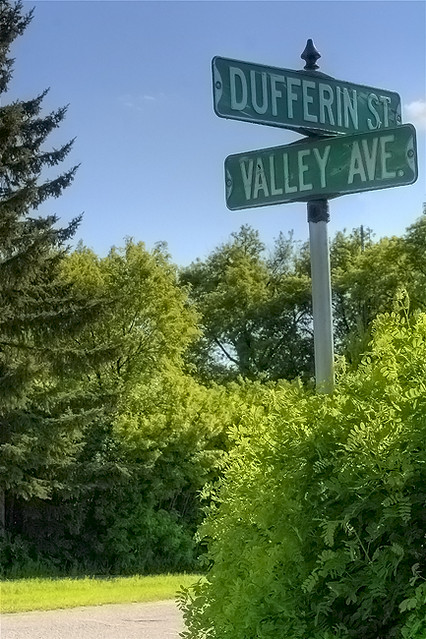In this photograph taken outdoors on a clear, midday, blue-sky day, a street sign featuring "Dufferin Street" and "Valley Avenue" stands prominently on a silverish-white pole at an intersection. Dufferin Street is displayed at the top on a green sign with bold white letters, slightly angled backward, while Valley Avenue sits below on another green sign, angled slightly forward, with a white decorative cap on either end. The top of the signpost is adorned with a small spear-shaped topper that flares out at the base, in dark gray or black. The bottom of the pole is obscured by a large leafy hedge, with a bush visible in the right corner. In the background, a tall pine tree occupies the left side of the image, stretching to the top edge, along with a mix of other lush green trees and bushes stretching across the frame. The lower left part of the scene shows a gray road and a patch of green grass. A tiny, delicate cloud appears to the right of the sign against the clear blue sky.